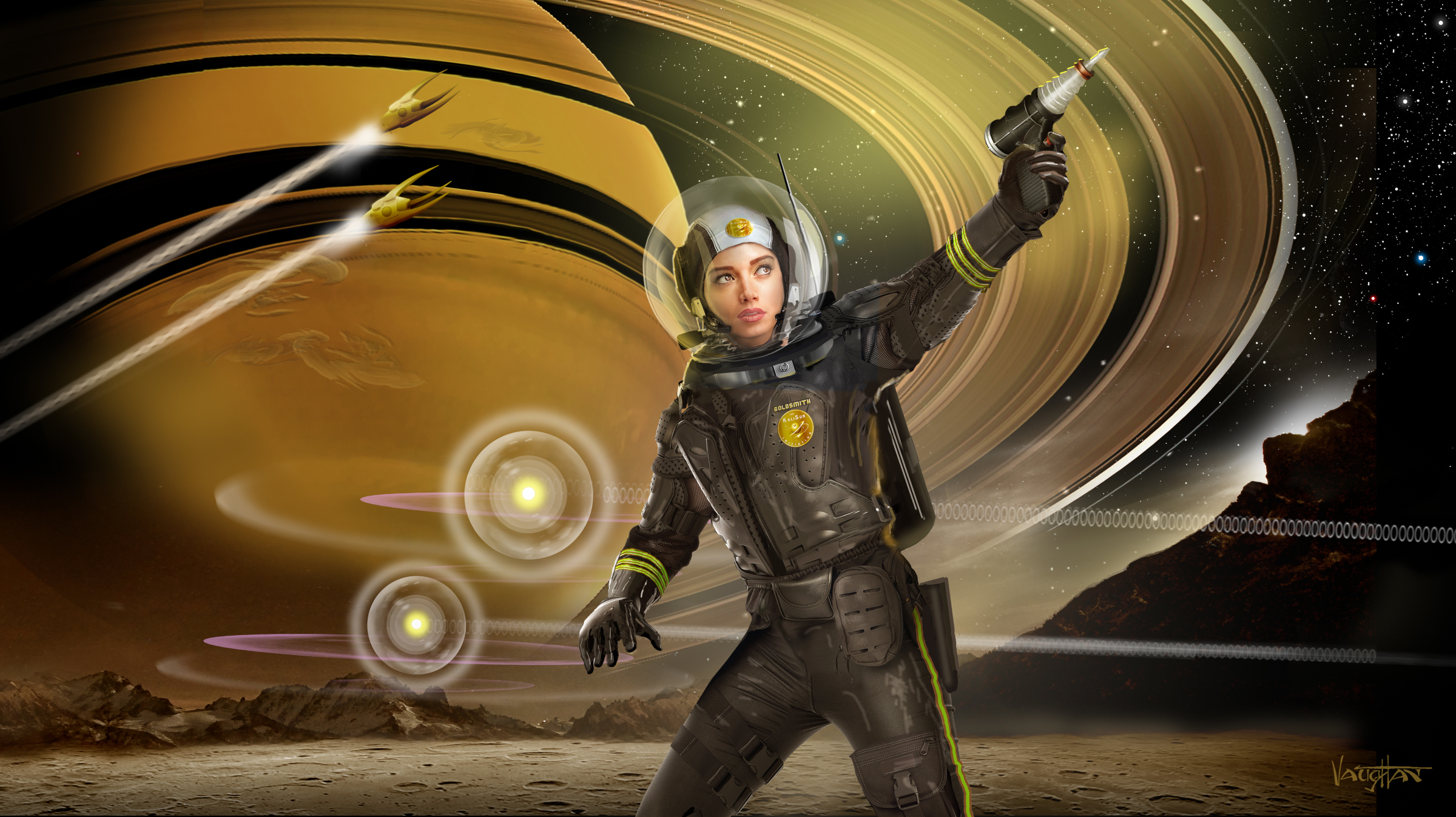In this detailed digital artwork, a young woman is depicted dressed as an astronaut in a tight-fitting, dark brown or gray spacesuit adorned with black gloves and accessorized with belts and knee guards. Her suit features yellow stripes around the wrists, and she wears a large, glass helmet with a white and black hat-like structure, possibly with an antenna on the back. In her left hand, she carries a ray gun.

The backdrop showcases a celestial landscape with flat, crater-strewn ground, hinting at meteorite impacts. To her right, there's a prominent rock formation. The black sky above is speckled with luminous stars and dominated by a giant, Saturn-like planet with glowing rings, occupying most of the view. Additional ringed planets glitter in the distance. 

Two yellow spacecraft, designed with three large spikes at their fronts, traverse the sky, leaving trails of white beams. The overall scene gives an impression of a moon-like surface with an ethereal, glowing quality, emphasizing a futuristic space exploration theme.